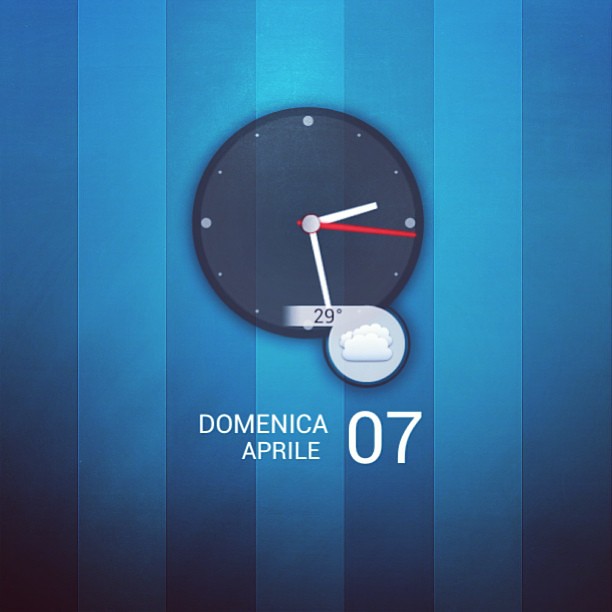A captivating animated image showcases a clock set against a striking dual-toned backdrop of dark blue and light blue stripes, evenly spaced in alternating fashion. The background consists of seven such stripes, providing a vivid contrast to the central clock. The clock is circular, featuring silver-colored markers for the hours of 12, 3, 6, and 9, with smaller silver dots denoting the remaining hours. Positioned near the bottom of the clock face is a smaller circle displaying puffy white clouds against a gray background, indicating a temperature of 29 degrees. Below this, white text provides location and date information: "Dominica, April 07." The clock itself has sleek white hour and minute hands, complemented by a contrasting red second hand, showing a precise time of 2:27 and 16 seconds.